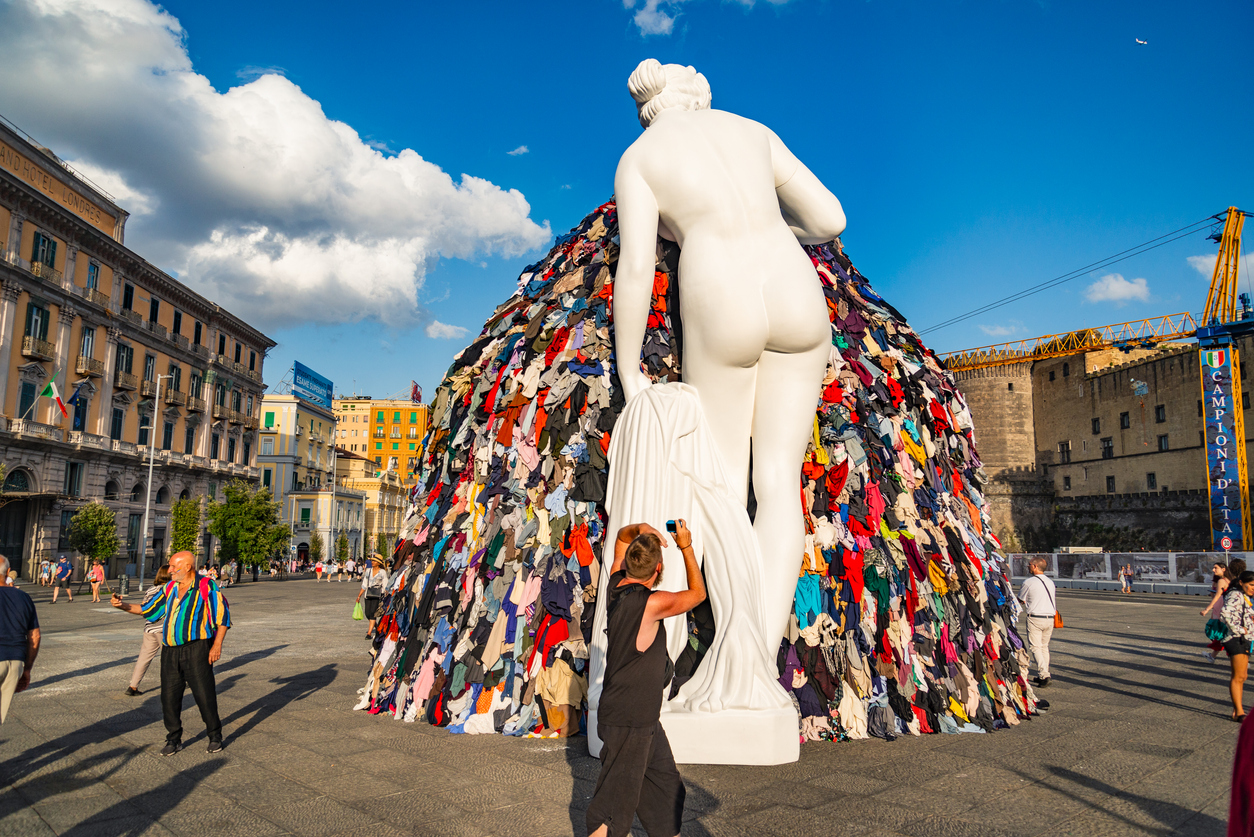This outdoor image captures a historical city square, surrounded by antique, low-rise buildings, evocative of an old-world architectural style. In the center of this open, cobblestone space stands an imposing, approximately 20-foot tall ivory statue of a naked woman. The statue, viewed from behind, depicts the woman leaning slightly forward, her hair styled in a low bun, and holding a sheet or robe in her left hand. She appears to be looking down at a large, triangular-shaped pile of colorful clothes, which may be around 15 to 20 feet high. The clothes encompass a wide spectrum of colors, including red, yellow, blue, white, off-white, cream, orange, green, and black. 

The scene is lively with approximately 30 people scattered throughout, some taking photos and others merely walking by. In the foreground, a woman in a brown dress shields her eyes from the sun while seemingly photographing the statue. To the lower left, a bald man wearing a multicolored tribal shirt is captured looking to his right. Another woman in shorts, wearing a backpack, appears on the right edge of the image. The background reveals a yellow building with green window shades on the left and a construction site with a banner that reads "CAMPIONIDITA" on the right. The day is partly cloudy, with a vivid blue sky enhancing the scene's vibrancy.